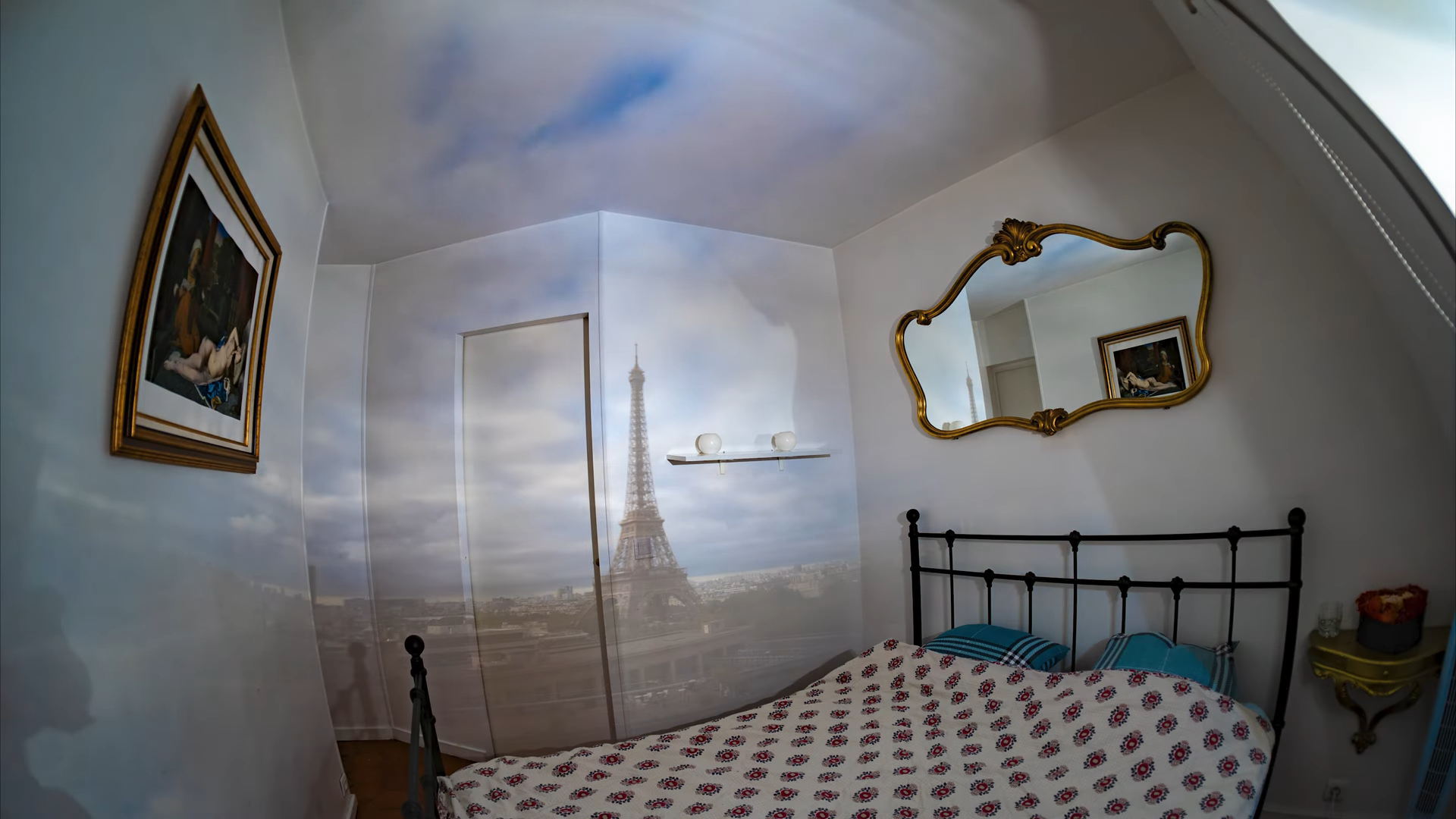This image depicts the interior of an older person's bedroom, possibly inside an apartment or condo. The room's odd angles suggest it might have been photographed with a fisheye lens. The focal point is a bed with a white comforter adorned with red flowers and pillows featuring blue geometric patterns. A sophisticated mirror hangs above the bed, reflecting the opposite wall where a Renaissance painting in a gold frame is displayed. The mirror and painting replicate a scene from Paris, including the Eiffel Tower, giving the impression of a wallpaper motif, with a blue and white cloudy sky adorning the ceiling.

To the right of the bed, a golden shelf attached to the wall holds a box with flowers and a glass of water. A nightstand sits beside the bed, although details are minimal. On one wall, there's a white shelf displaying two round pots or ceramic pieces and a door. The room's color palette incorporates shades of blue, white, pink, and gold, which adds to the antique ambiance. The walls are peculiar in shape, giving the room a uniquely angled structure. While the room primarily features old-fashioned elements, the overall decoration suggests a nostalgic charm.